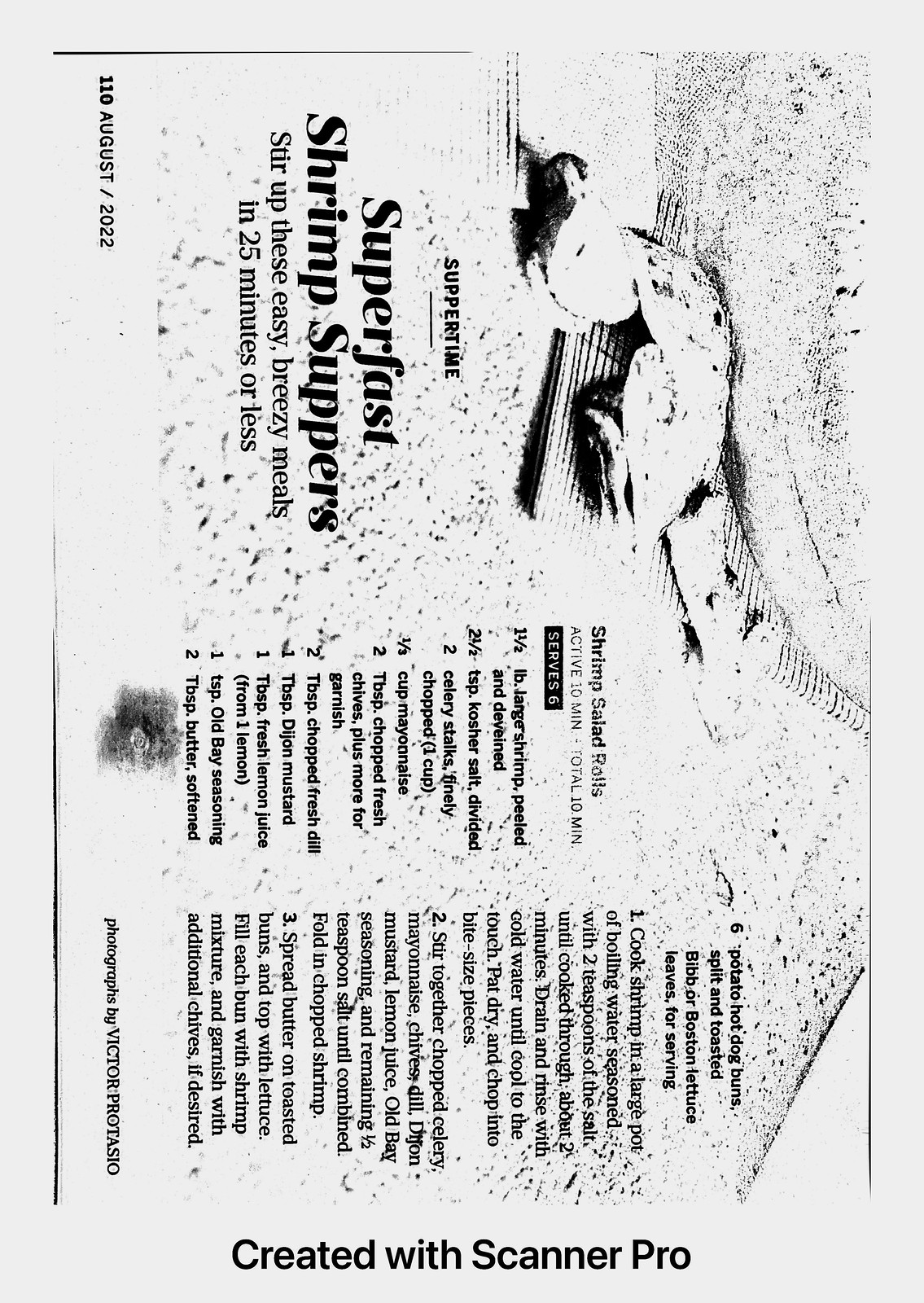This detailed black and white scanned image, taken from what appears to be a page in an old magazine or book, captures a recipe for "Super Fast Shrimp Suppers." The background is light gray, and the image orientation requires you to turn it sideways for proper reading. Across the top in intricate black text, it announces: "Suppertime: Super Fast Shrimp Suppers. Stir up these easy breezy meals in 25 minutes or less."

The highlighted recipe is for "Shrimp Salad Rolls," catered to serve six. The preparation and cooking times are remarkably swift, with active cooking time listed as 10 minutes. The recipe begins with cooking 1.5 pounds of large shrimp, peeled and deveined, in a large pot of boiling water seasoned with two teaspoons of kosher salt until cooked through, approximately two minutes. 

The subsequent steps include stirring in finely chopped celery, mayonnaise, Dijon mustard, fresh lemon juice, Old Bay seasoning, and herbs like chives and dill. For serving, the shrimp salad mixture is filled into toasted potato hot dog buns that have been buttered, with bib or Boston lettuce leaves added for extra crunch. 

Further details identify the scanner used—Scanner Pro—and the image credits, indicating it was photographed by Victor Protasio and originally found on page 110 of an issue dating to August 2022. The grainy image includes an indistinguishable object that vaguely resembles a turtle going down a road, adding to the rustic, monochrome charm of the scanned page.